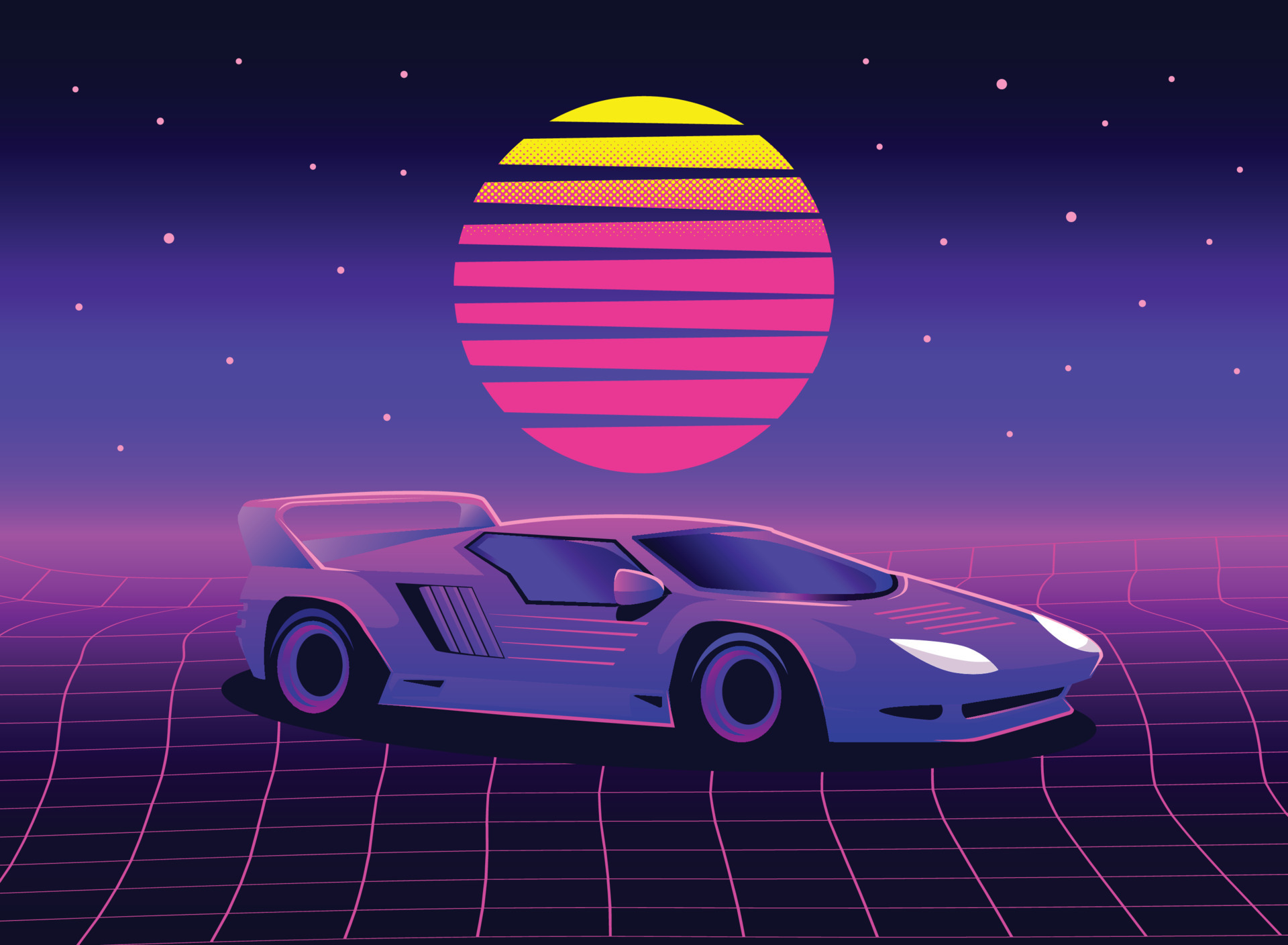The illustration is a striking digital depiction exuding strong 1980s retro-futuristic vibes. Central to the image is a sleek, cartoonish sports car, reminiscent of classic Lamborghinis or Ferraris, yet distinctly unique. The car features a two-tone color scheme with a purple lower body and a pink upper body, complemented by big black wheels with pink inner rims and a prominent pink and purple rear wing. The car faces right, showing off its design that hints at high speed and luxury.

Set against a vibrant, gradient sky, the scene captures the essence of a sunset transitioning from pink at the bottom to bright yellow at the top, with streaks cutting through the sun allowing glimpses of the background. The sky transitions from light blue near the horizon to almost black at the top, dotted with star-like specks. The futuristic landscape is anchored by a grid-patterned floor, dark with pink lines that curve towards the car, akin to a Tron aesthetic.

Overall, the image brilliantly blends elements of synth-wave and sci-fi, creating a visually captivating homage to the electronic 1980s era.